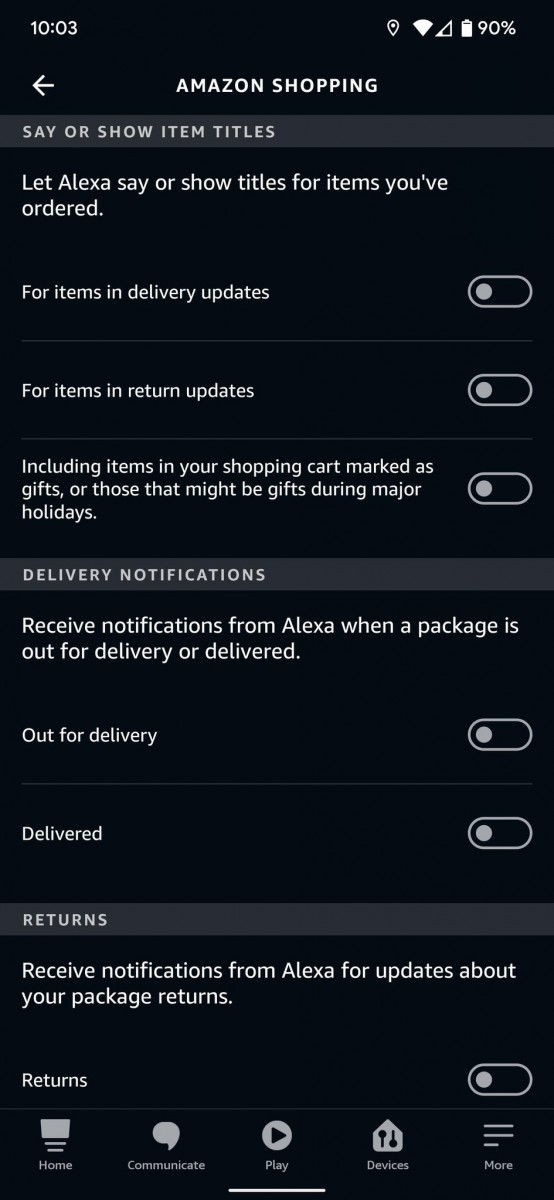This is a detailed screenshot of a mobile phone displaying the Amazon Shopping app with a dark background. 

In the top left corner, the time is shown as "10:03" in white text. Adjacent to it on the right, the battery indicator displays "90%," followed by icons indicating the Wi-Fi signal strength as full, a low cellular signal with one bar, and an active location service.

Centered at the top, in bold white capital letters, is "AMAZON SHOPPING." Beneath this header is a thin dark gray line containing the phrase "SAY OR SHOW ITEM TITLES" in white, all capital letters.

Following this, there's a message on a black background stating: "Let Alexa say or show titles for items you've ordered." This text is split into two lines. Below this, it mentions, "For items in delivery updates," with a toggle switch on the right side indicating the feature is turned off.

Further down on the left side, it says "For items in return updates," with its respective toggle switch turned off on the left side. The next line reads, "Including items in your shopping cart marked as gifts, or those that might be gifts during major holidays." This feature is also toggled off to the right.

A thin gray border separates these sections, below which "DELIVERY NOTIFICATIONS" is written in all capital white letters. Beneath this section, against a black background, the text reads: "Receive notifications from Alexa when a package is out for delivery or delivered."

Further details include a subsection where "Out for delivery" is mentioned on the left with the toggle switch turned off on the right, and "Delivered" also on the left with a toggled-off switch.

Next, there's a gray bar labeled "RETURNS," followed by a message on a black background that reads: "Receive notifications from Alexa for updates about your package returns." The associated toggle switch for "Returns" is also turned off.

At the very bottom, a navigation bar shows icons for "Home" on the left, "Communicate," "Play" in the center, "Devices," and "More" on the right.

Each toggle switch has a grey border with the circle inside noted as grey, indicating that all functions are currently deactivated.